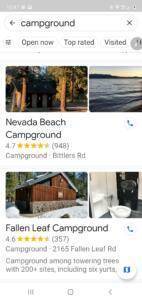The image in question appears to be a screenshot of a mobile device, though the quality is exceptionally low. It's highly pixelated and marred by numerous JPEG artifacts and blurred images. Text throughout the image is similarly blurred, obscuring details such as the time and battery life in the status bar at the top. The application or platform being used is indeterminable, but it depicts a search results page focused on campgrounds.

At the top of the screen, there are filter options such as "Open Now," "Top Rated," and "Visited." Two campground listings are partially visible, each accompanied by two images that generally depict open and natural outdoor scenes.

The first listing is for the "Nevada Beach Campground," boasting a rating of 4.7 stars based on 948 reviews. The text indicates that this campground is located on a road whose name is unclear due to the image quality—possibly "Bitters Road," "Battles Road," or something similar.

The second listing is for "Fallen Leaf Campground," with a rating of 4.6 stars from 357 reviews. Its address is listed as 2165 Fallen Leaf Road. The description states that it is a "campground among towering trees with 200 plus sites including," though the final part of the sentence is difficult to discern, seeming to suggest the inclusion of six yurts.